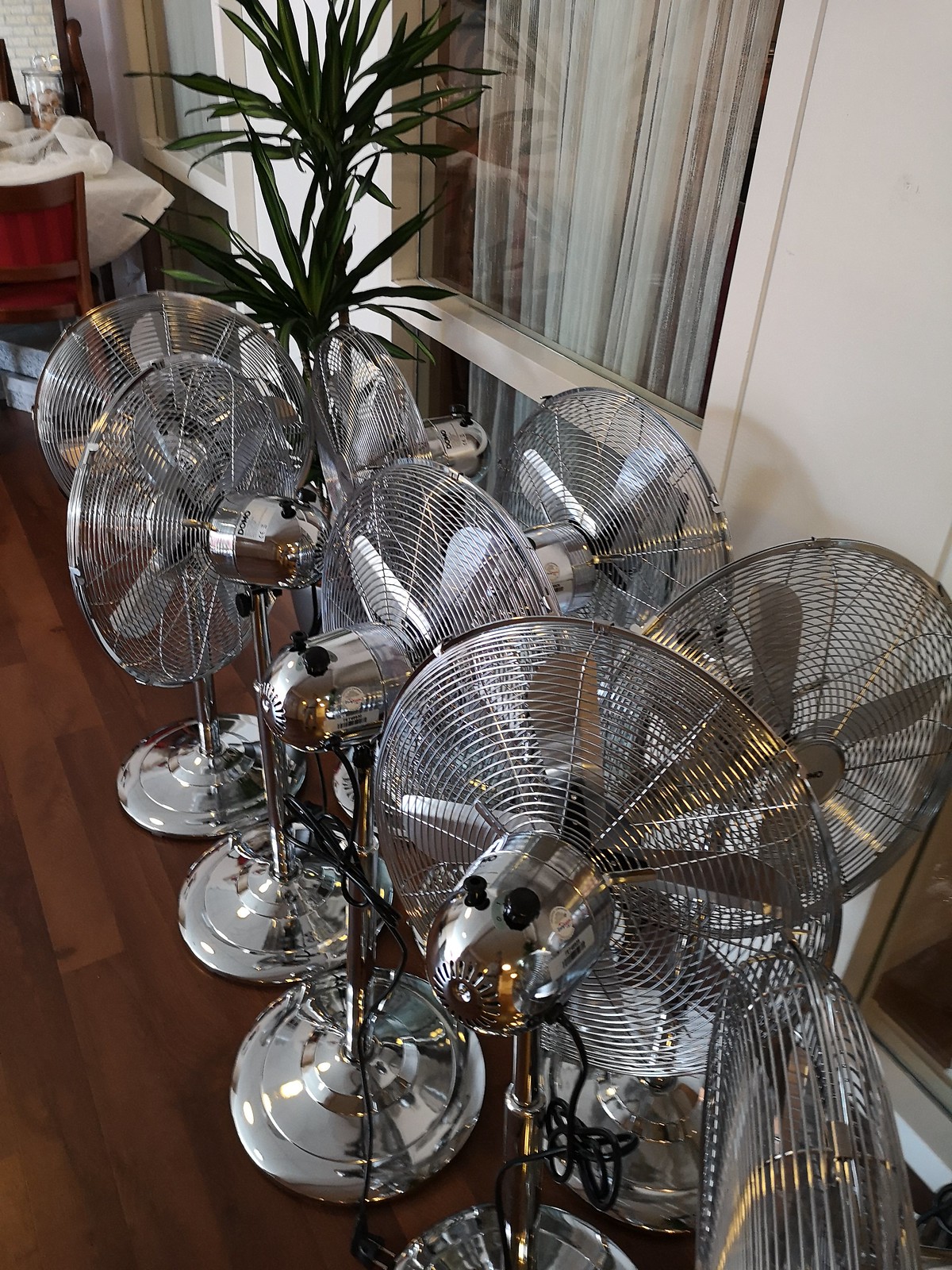In this photograph, a set of eight stainless steel standing fans are organized in two rows on a polished, dark reddish-brown hardwood floor. Each fan boasts a high-polished circular base, a sturdy metal support rod, and a rounded fan head encased in a silver mesh cover with multiple blades inside. The fans feature black electric cords and black control buttons located on their back panels. In addition to the fans, a potted plant with thin, long, dark green leaves, resembling a palm tree, stands to the left. This setup is placed in front of a large, glass-paned window that is divided into a top and bottom half, bordered by a white painted frame. Behind the glass, there are thin white curtains. The window is set into a white paneled wall, adding to the room’s clean aesthetic. In the background, positioned in the top left corner of the frame, a wooden dining table covered with a white tablecloth and accompanied by a single red-brown wooden chair can be seen, adding a touch of cozy home decor to the scene.